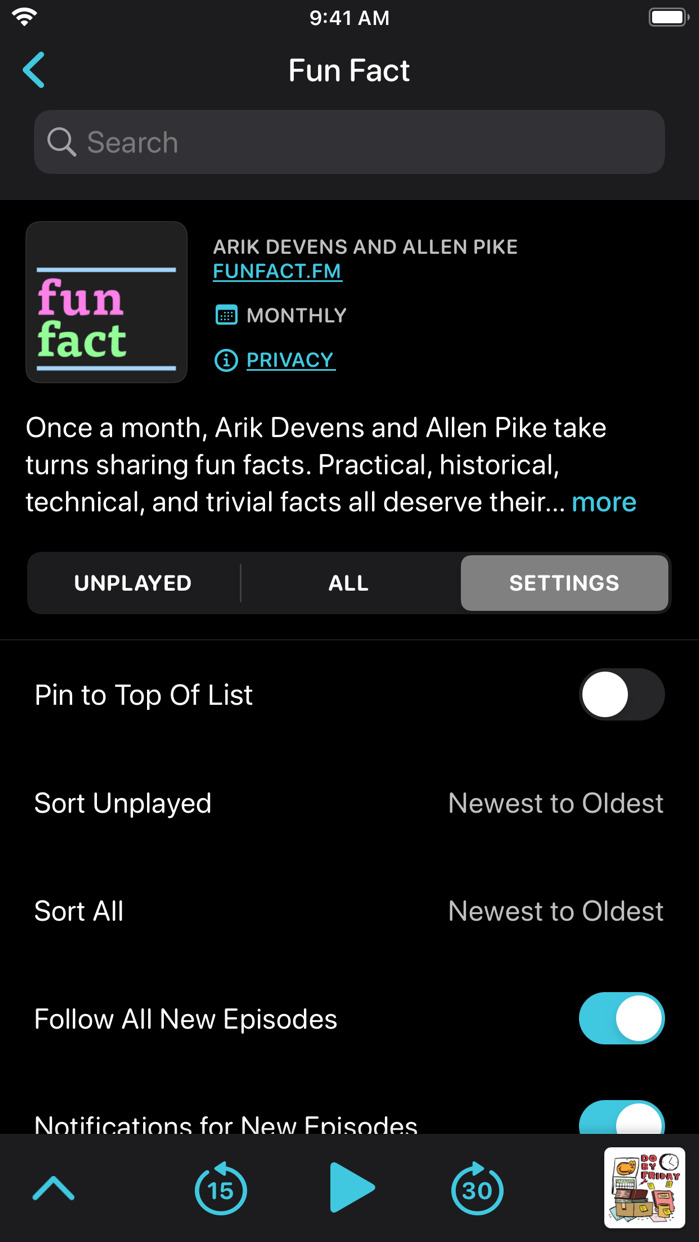This image depicts a phone application screen in portrait orientation, characterized by its black background and white text, with interactive elements highlighted in teal. At the very top of the screen, the time is displayed as 9:41 a.m. on the left, a Wi-Fi signal icon in the center, and a battery indicator on the right. Below this header, a search bar is prominently positioned under the words "Fun Fact." 

Directly beneath the search bar, there's a colorful logo that features the word "Fun" in vibrant pink and "Fact" in a striking lime green. Adjacent to this logo, the app displays the name of the user, a frequency indicator, and privacy settings options.

Continuing down, a detailed description of the service provided by the app is presented. At the bottom of the screen, a horizontal navigation bar features three selectable options: "Unplayed" on the left, "All" in the center, and "Settings" on the right. Users can tap on any of these options to filter and view content according to the selected category.